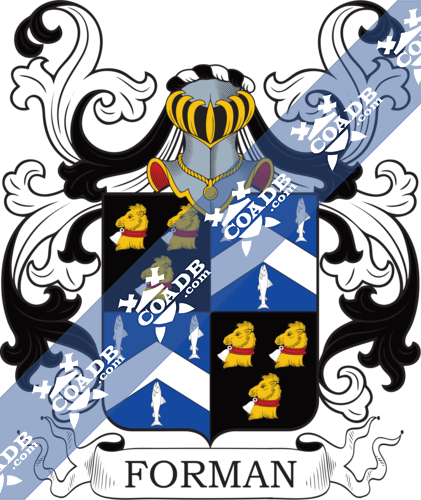The image depicts an intricate coat of arms for the Foreman family. The top section features an ornate crest resembling a neck adorned with a gold necklace and a medallion. The background of the crest has a black and white paisley design spreading outward. Below the crest, there is a shield divided into four quadrants. The top left and bottom right quadrants feature a black background with a gold cow and cowbell. The top right and bottom left quadrants display a blue background with three white fish. The shield is encompassed by elaborate black and white decorative frills. A scroll beneath the shield reads 'Foreman' in black font. Overall, the design combines elements like a knight's helmet with yellow gold accents and intricate details, emphasizing the complexity and heritage of the Foreman coat of arms.